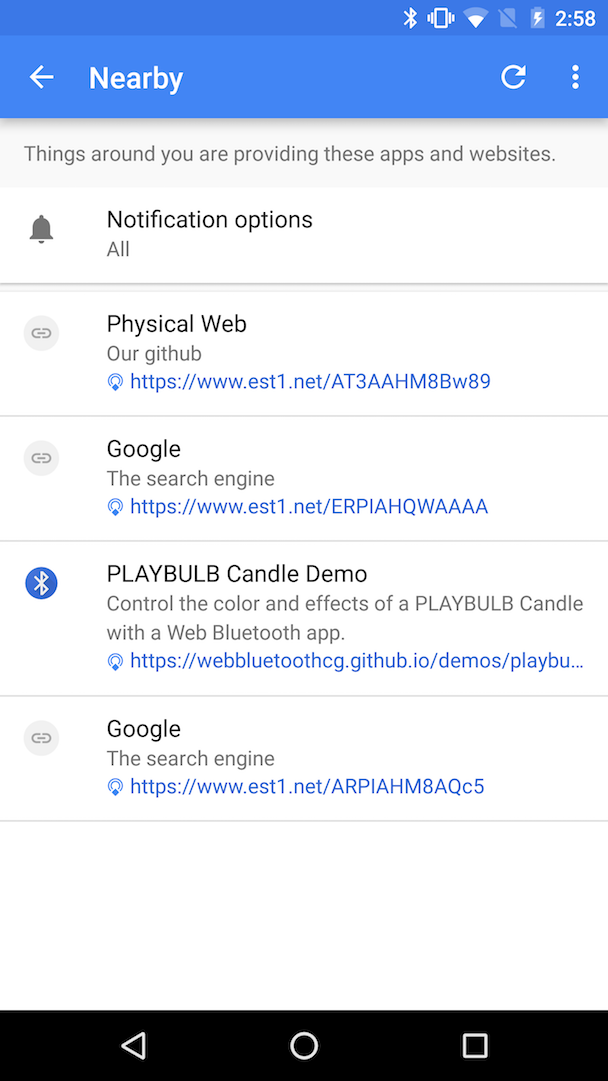This is a detailed screenshot of a mobile device interface depicting a variety of system icons and informational content. At the top of the image is a blue status bar showcasing several white icons, including a Bluetooth symbol, a cell phone icon with signal waves, a Wi-Fi icon, a square icon with a diagonal slash, and a battery icon with a lightning bolt, indicating it's 2:58. 

Below, a white back arrow labeled "Nearby," a white refresh arrow, and three white dots are visible. The main section below this displays a white background with blue and gray text that reads: "Things around you are providing these apps and websites." Additionally, there's a bell icon labeled "Notification Options All." A paperclip icon is followed by "Physical Web, our GitHub," accompanied by a blue hyperlink.

Further down, another paperclip icon titled "Google the search engine" appears with a blue hyperlink. An adjacent section shows a blue and white Bluetooth symbol with the text "Play bulb candle demo" in black. This section also explains, "Control the color and effects of a PLAYBULB candle with a web Bluetooth app," alongside another blue hyperlink. Below this, once more, a paperclip icon and the label "Google the search engine" with a blue hyperlink are presented, each hyperlink featuring an icon resembling a person with lines above their head.

At the bottom of the screenshot, a black navigation bar is visible, containing a white back arrow, a white circle, and a white square.